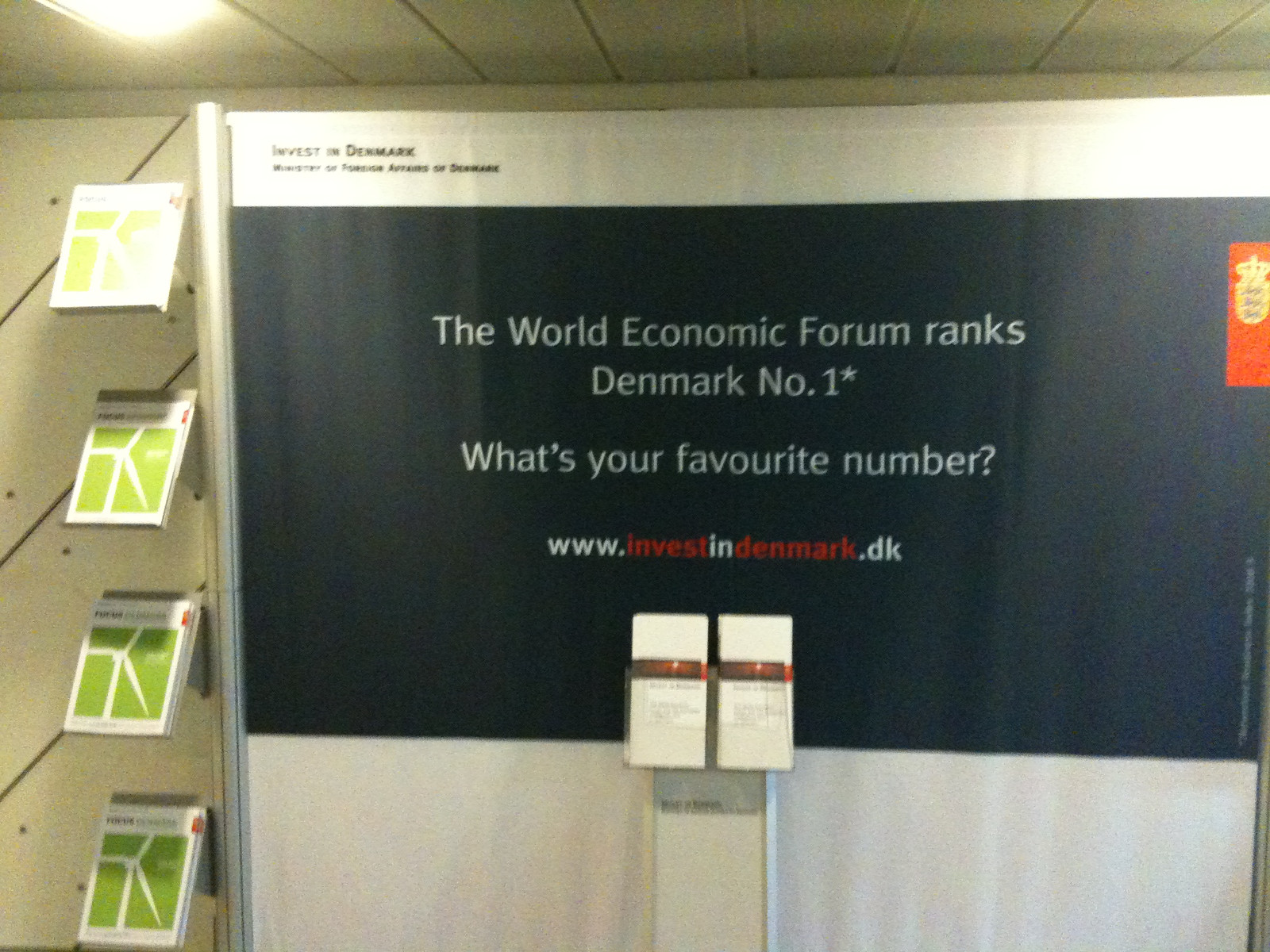The image depicts a somewhat grainy and poorly lit brochure setup, likely taken inside an office building. The main focal point is a large promotional panel featuring a dark blue background with the text "Invest in Denmark" at the top in white. Below it, also in white text, it reads, "The World Economic Forum ranks Denmark number one. What's your favorite number?" The URL "www.investindenmark.dk" is displayed beneath the text, with "Invest" and "Denmark" highlighted in red.

In front of this main panel, a stand holds multiple smaller brochures, suggesting promotional material related to Denmark. To the left of the panel, there is another rack containing more brochures, some of which feature images of windmills. An additional small orange block is present in the upper right-hand corner of the panel. Overall, the scene aims to encourage investment in Denmark, despite the image's somewhat blurry and greenish cast due to inadequate lighting.